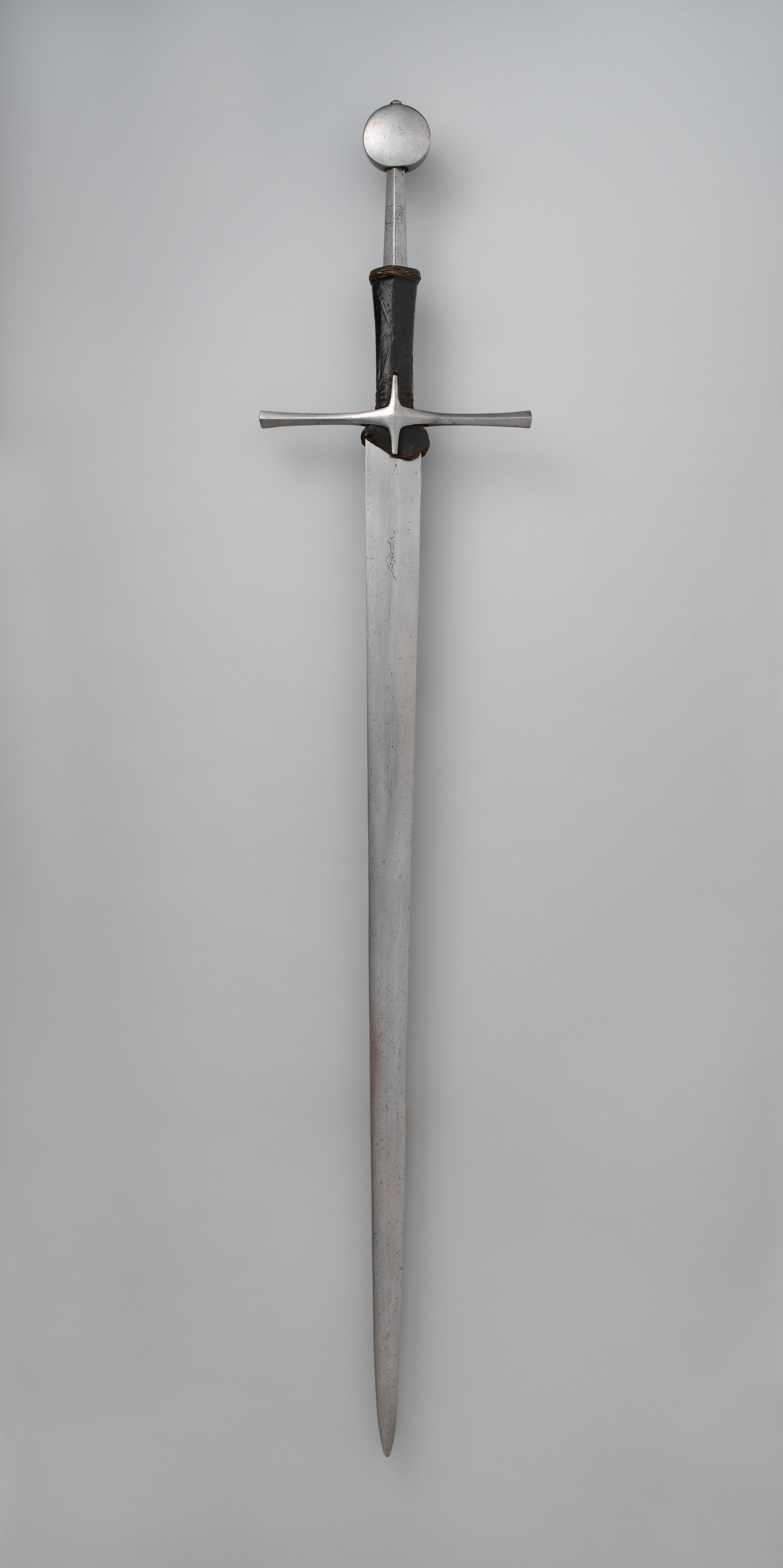The image is a detailed photograph of a modern-looking sword, captured in a rectangular portrait orientation. The sword, centrally positioned against a light gray background, appears almost suspended, casting minimal shadows, suggesting it is either hanging or the image is AI-generated. The sword itself is predominantly silver, exhibiting a highly polished, reflective surface. From the top, the handle features a round, silver pommel, resembling the shape of a steel lollipop. The handle is wrapped in black leather, offering a striking contrast to the metallic sheen. Just below this black grip is a thin crossguard, or horizontal piece, extending like a plus sign or a four-pointed starburst in metal. The blade is straight and narrow, uniformly tapering to a sharp point. The image contains fine details like subtle shadows reflecting the light in a way that merges the blade slightly with the background, enhancing the sleek, streamlined aesthetic of the sword.